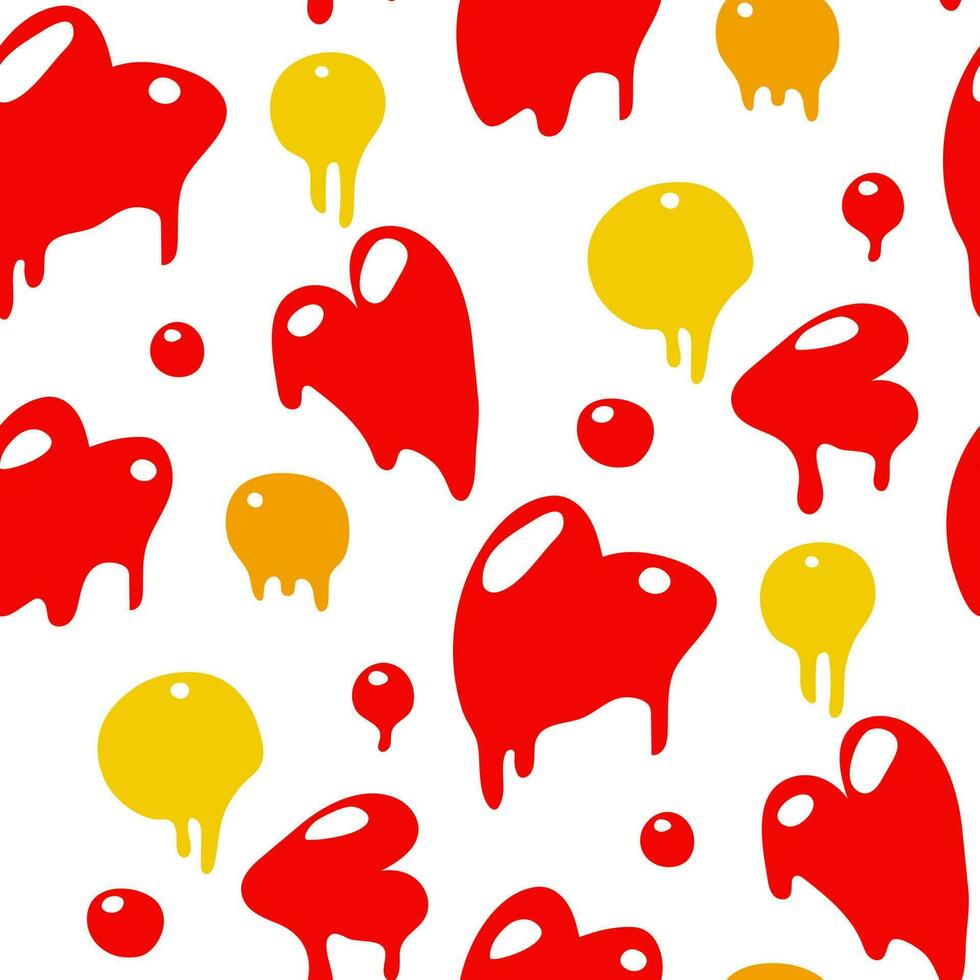The image is a computer-generated graphic with a predominantly white background, featuring a repetitive pattern of various colorful objects. Central to the design are nine red hearts, which appear to be dripping as if they were made from melting red paint. These hearts, which face random directions, each have two white spots resembling reflections. Complementing the hearts are five uniformly colored circles that range from yellow to orange, which also have white reflection spots and appear to be dripping. Additionally, there are six smaller red dots dispersed throughout the image; while some of these dots exhibit a dripping effect, not all do. The overall pattern is evenly distributed and creates a striking visual contrast against the white background.